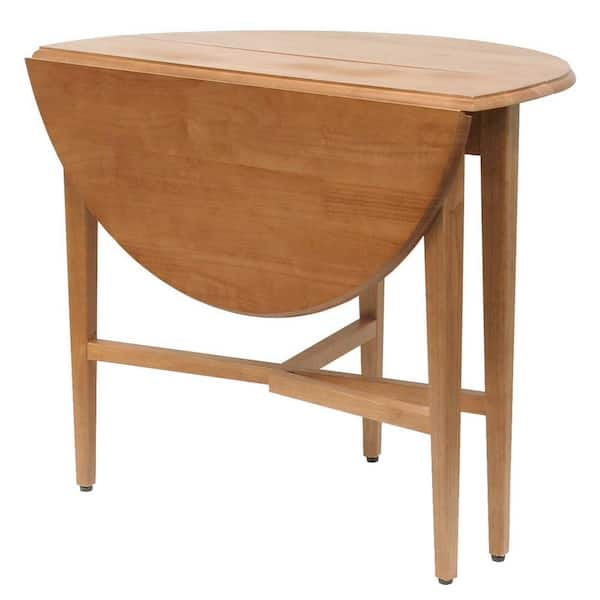This photograph showcases a versatile, mid-century style wooden table, designed to adapt to various needs. When fully opened, the table features a round top, perfect for several chairs, and is composed of medium-colored, unfinished maple or oak wood with beveled edges. The table's distinctive design includes hinges that allow the tabletop to fold, transforming it from a round shape to a half-moon or a narrow rectangular table. Each of its four legs, equipped with small stoppers to protect floors from scratches, cleverly aligns next to one another as the table is folded, ensuring compact storage. This multifunctional table, notably simplistic in design, can serve as a full dining piece, a handy half-table, or even a small side table behind a sofa, making it a highly convenient piece of furniture.